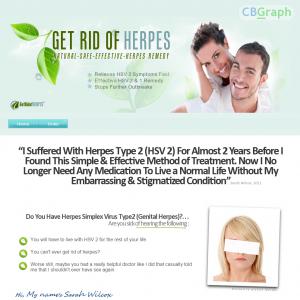**Caption for Image:**

The image prominently features an advertisement for a CBG graft, a natural remedy claimed to eliminate herpes. The phrase "Get Rid of Herpes" is highlighted in green text. Surrounding the main text are illustrations of mint leaves, underscoring the natural aspect of the product. Underneath, it reassures potential users with the words "Natural, Safe," implying accessibility and affordability. The image showcases a happy couple, suggesting the remedy's effectiveness in improving their lives. At the bottom of the image, there are two small, blue buttons with text that is not legible due to its size.

Adjacent to the main image is a testimonial from a user who suffered from HSV-2 for nearly two years before discovering this effective treatment. The user, a fair-skinned blonde woman with partially covered face and visible eyes, shares that she no longer requires medication to manage her condition and can lead a normal life free from the stigma of herpes. The quote is paired with a call-to-action inquiring about the viewer's own herpes status, accompanied by green buttons encouraging further exploration of the remedy.

**Note:** The text indicates a strong message of hope and relief for individuals affected by herpes, urging them to click for more information about this promising treatment.